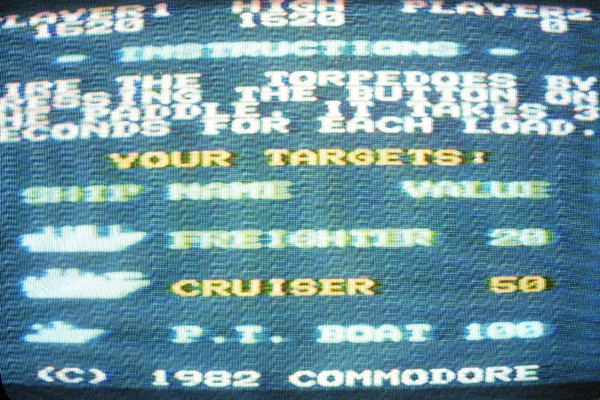This image is a slightly blurry photograph of a TV screen displaying a portion of a 1982 Commodore video game. The screen, likely from a tube TV, shows slightly curved edges, contributing to the nostalgic feel. Across the top portion of the image in large white text, it reads "PLAYER ONE," "PLAYER TWO," and "HIGH SCORE." Below this, yellow text instructs players to "USE THE TORPEDOES" and identify "YOUR TARGETS," although some of this text appears blurry and difficult to decipher. Further down, also in yellow text, it lists "CRUISER 50" as one of the targets. The background is a grainy bluish-green color, characteristic of early video game graphics. At the bottom of the image, in white text, it states "COPYRIGHT 1982 COMMODORE," underscoring the vintage nature of the game.